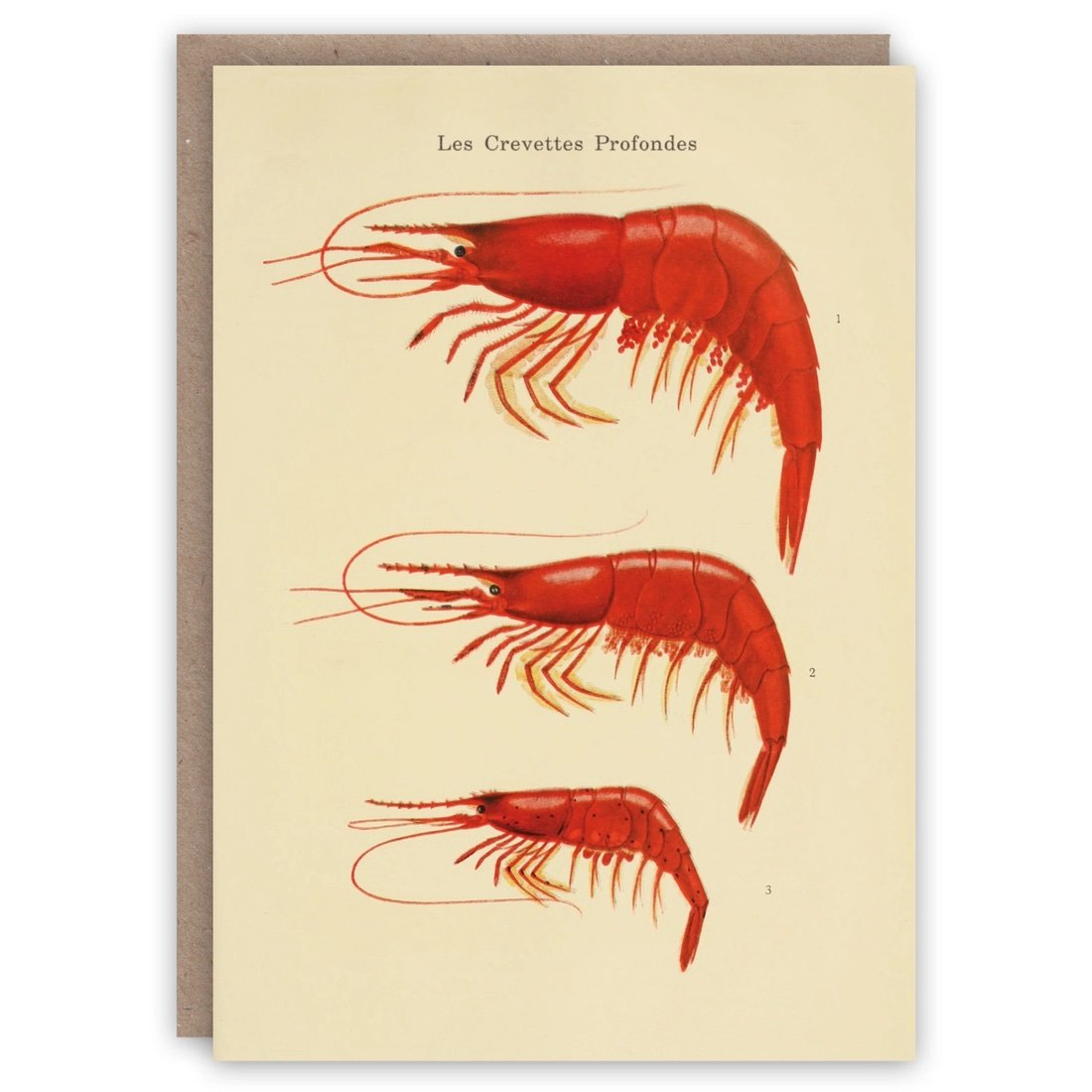The image displays a detailed, hand-drawn illustration of three shrimp, labeled "Les crevettes profondes" at the top in dark text. Each shrimp is intricately drawn with a red shell and multiple legs, with antennas extending from their heads. The shrimps are stacked vertically, with the largest on top, a medium-sized one in the middle, and the smallest at the bottom. Notably, the shrimp at the bottom distinguishes itself with black spots across its shell. The entire illustration is set against a yellowed white paper, which is placed on top of an identically sized piece of recycled brown cardboard, giving it a framed appearance.